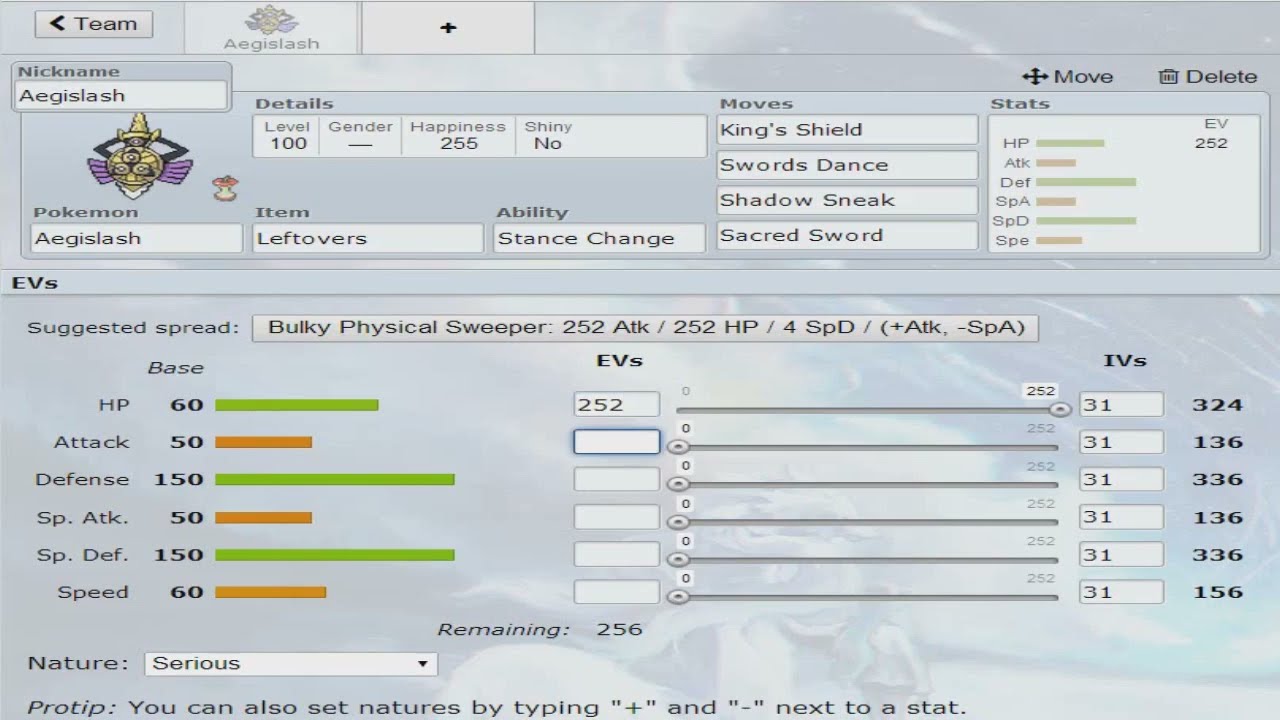The image appears to be a detailed screenshot from a Pokémon application or game interface dedicated to the Pokémon Aegislash. At the top left, it prominently displays "Team" with an arrow to the left and a partially translucent profile tab. Across the screen, Aegislash's information is meticulously laid out. The Pokémon is represented by an image featuring a yellow shield with dots, arm-like appendages, purple wings, and a small white dome. Key details include the nickname "Aegislash," level 100, gender unspecified (indicated by a dash), happiness at maximum (255), and a non-shiny status. Its ability is "Stance Change." The moves listed are King’s Shield, Swords Dance, Shadow Sneak, and Sacred Sword. The interface also displays a stats section with horizontal bars showing values for HP, Attack, Defense, Special Attack, Special Defense, and Speed, with colors ranging from red to green to indicate different levels. Below, there is a section titled "Usable Moves," listing Aerial Ace, Autotomize, Brick Break, Destiny Bond, Facade, Flash Cannon, Frustration, and Gyro Ball. The overall design suggests this is an application for managing and viewing detailed Pokémon statistics and capabilities.